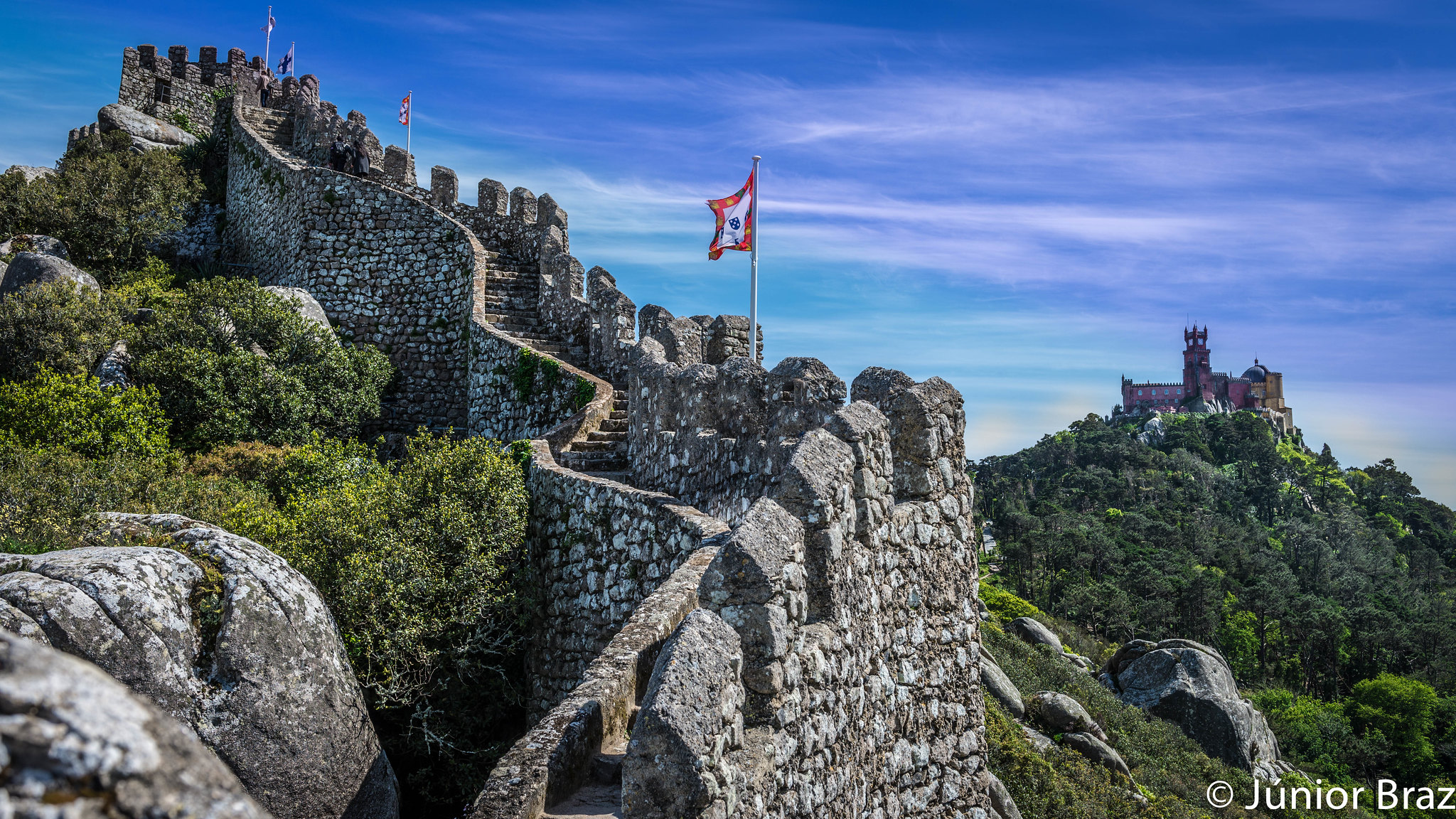A breathtaking view of Cusco, featuring the Junior Brass Monolith set against a spectacular, deep blue sky dotted with white clouds. The scene is dominated by a robust stone wall that winds from the foreground, snaking its way up toward the tallest tower of an ancient castle or manor in the distance. Red flags are prominently posted along the wall, adding a splash of color to the stone structure. The hillside is adorned with various shades of green leaves and grass, with some rocks peeking through the verdant landscape. The overall composition captures the timeless beauty and historical richness of the area.